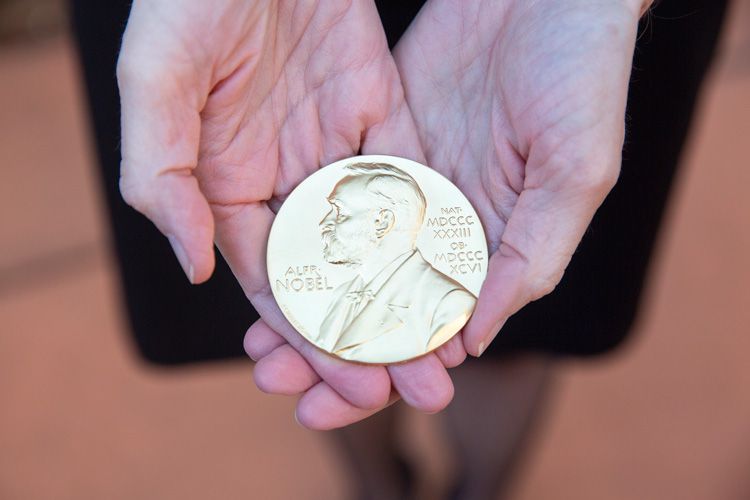The image depicts a detailed and shiny gold Nobel Prize medal held in the cupped, wrinkled hands of an elderly Caucasian woman. The medal features a side profile engraving of Alfred Nobel, who is bearded with short hair, wearing a suit and bow tie, and facing left. The inscription "Alfred Nobel" is visible on the left side of the medal. Below his name are Roman numerals: "Nat MDCCC," "XXXIII," "OB," "MDCCC," and "XCVI" sequentially stacked. The photograph is taken from above, revealing part of the woman’s legs, clad in black stockings, and the indistinct, blurry backdrop has a faint orangish-pink hue. The woman's dress is dark, contributing to the background's overall dim ambiance.